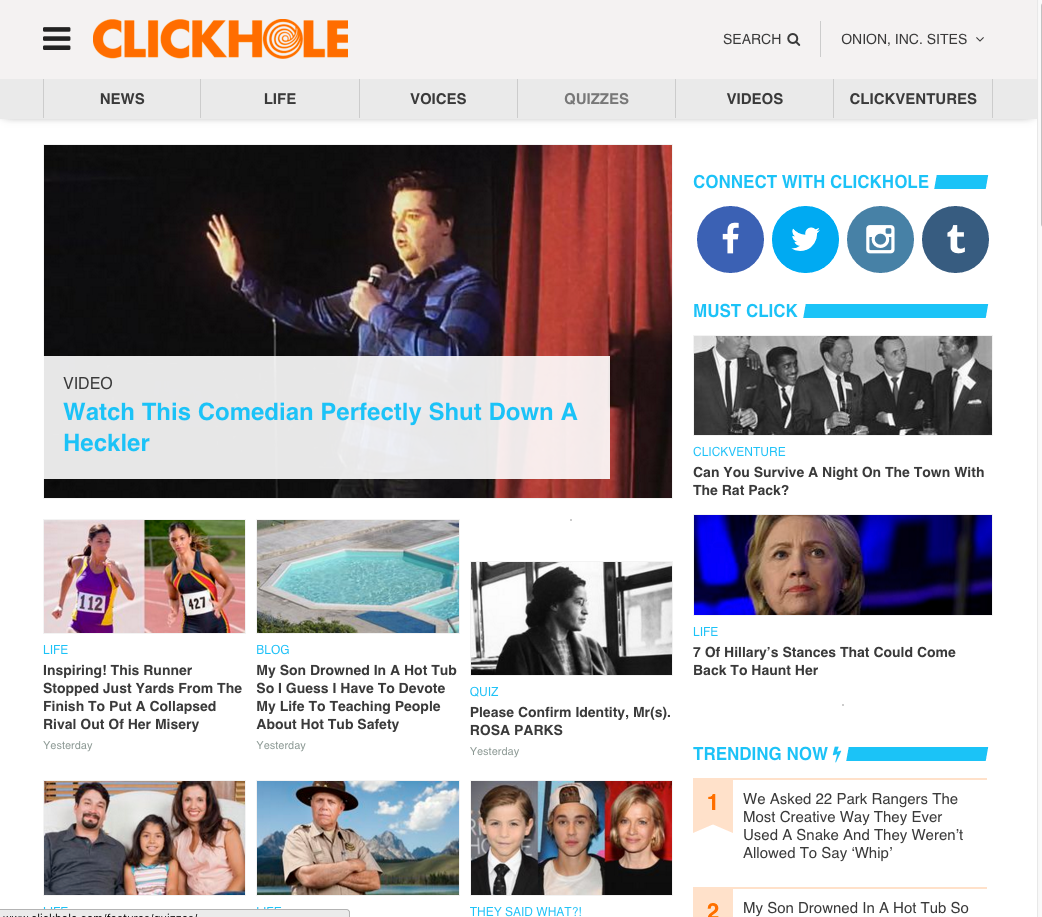The image is a web screenshot displaying a quizzes screen from the website ClickHole. The ClickHole logo is prominently placed in the upper left corner, rendered in capital letters with orange text, and features a spiral design within the "O." To the left of this title are three vertical lines on a light gray banner. In the upper right corner, there is a search icon and a drop-down menu for Onion, Inc. sites.

Six main headings are visible: News, Life, Voices, Quizzes, Videos, and ClickVentures. The Quizzes tab is highlighted, indicating the current section being viewed. The upper left area of the page showcases a video titled "Watch this comedian perfectly shut down a heckler," with an image of a comedian on stage in a blue plaid shirt.

Beneath the video, there are six sections featuring photographs, labeled Life, Blog, and Quiz. The screenshot cuts off part of the bottom left section, while a vertical column runs along the right side. The first section in this column is titled "Connect with ClickHole" and includes four social media icons. Below this, a "Must Click" section contains two horizontal images labeled ClickVenture and Life. In the bottom right corner, the "Trending Now" section lists two trending items, denoted as number one and number two, accompanied by black text descriptions.